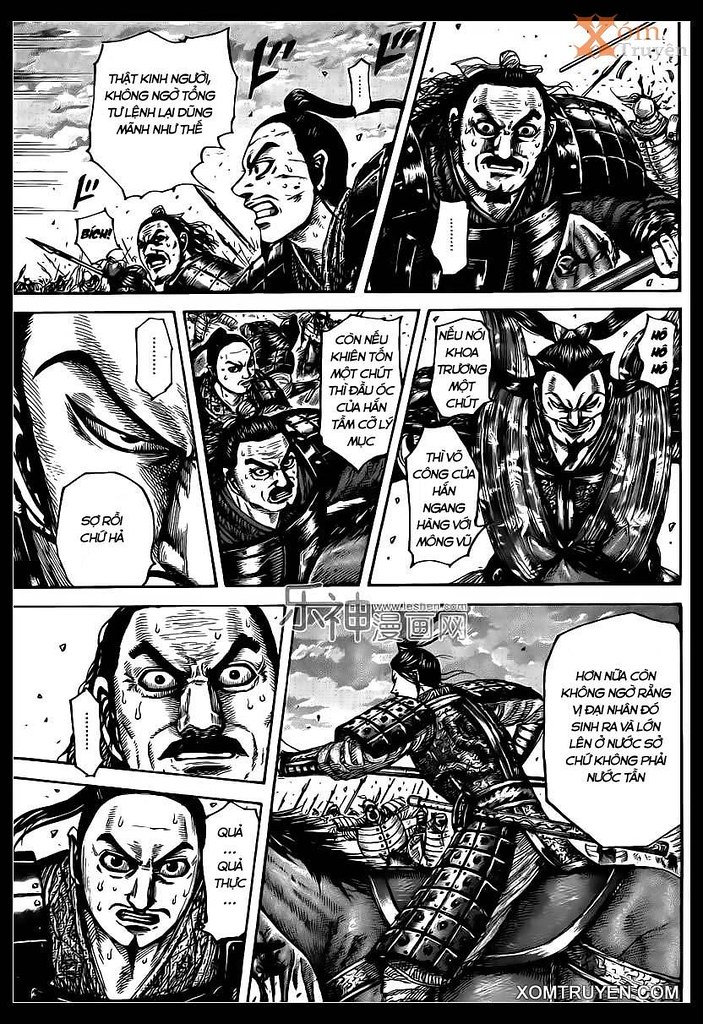This is a highly detailed black-and-white page from a graphic novel, resembling a cartoon, set in the middle of a battlefield involving samurai warriors. The page consists of eight distinct panels framed by thin black lines. The top row features two panels: the left one shows warriors charging into battle, while the right one depicts a warrior seemingly charging towards the viewer. The second row contains a close-up of a warrior's eye on the left, two warriors in combat in the middle, and a single warrior looking down, facing the viewer on the right. The bottom row has a sweating warrior glaring intensely in the panel on the left, which transitions to another image of the same warrior from a slightly farther perspective, still showing sweat and intense focus. The final panel on the bottom right captures the warrior on a horse, heading left. The text at the bottom spelled out "XOM TRUYEN COM", and the characters are speaking in an unfamiliar, likely Asian language. The scene clearly depicts an intense battle, with warriors in armor equipped with swords, some riding horses, all exhibiting expressions of aggression typical of a combat situation.